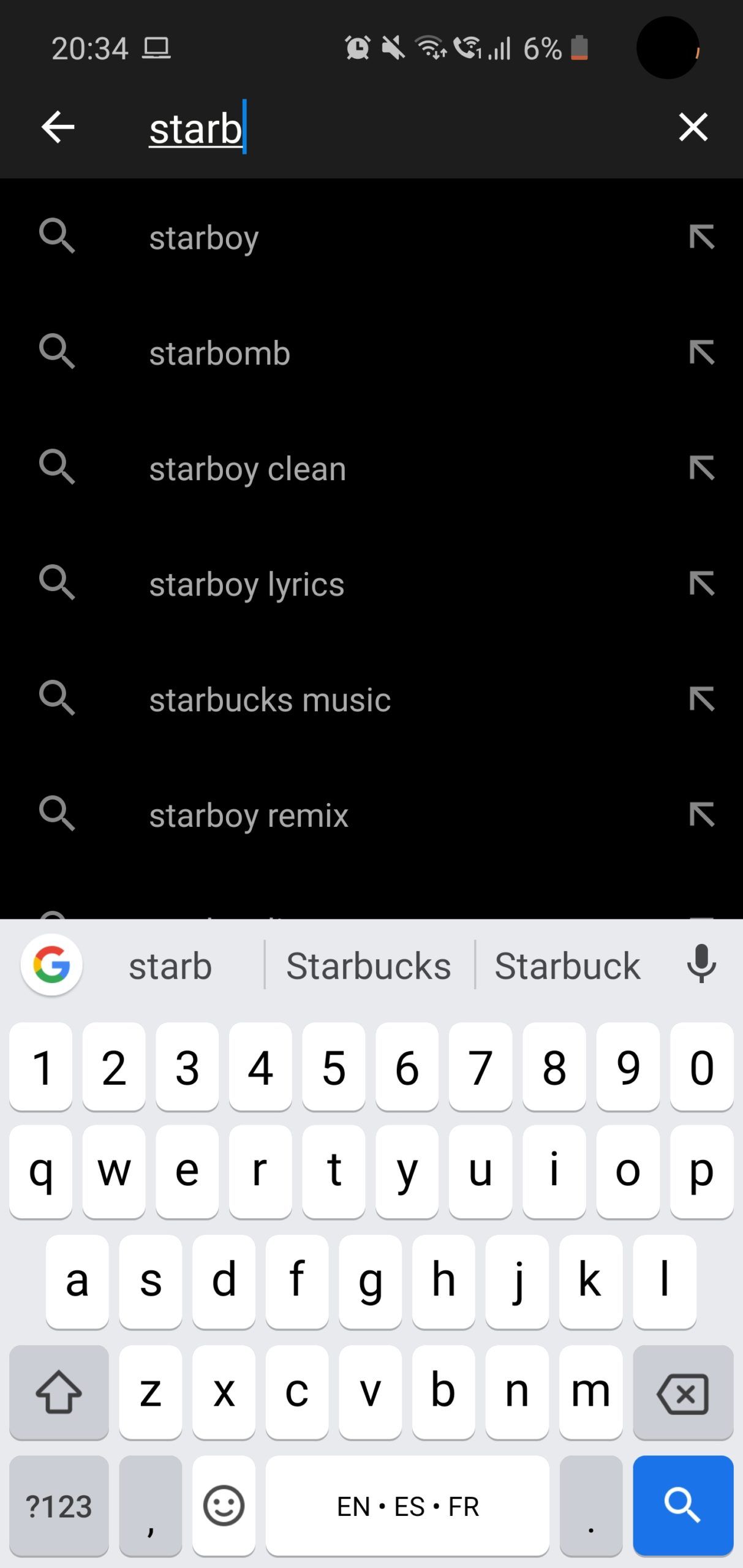The image is a screenshot of a smartphone's search bar interface. At the very top, there is a black rectangular area. An arrow pointing to the left is visible within this rectangle. Below the black rectangle, the search query field displays the partially typed word "STARB" followed by a vertical blue line, indicating the cursor's position.

Suggestions related to the typed query appear underneath the search field: "Starboy," "Starbomb," "Storyboy Clean," "Starboy Lyrics," "Starbucks Music," and "Starboy Reef Mix." Below these suggestions, the Google logo, a circle containing the letter 'G,' is prominently displayed.

The bottom portion of the screenshot showcases the virtual keyboard. The QWERTY layout is visible, complete with rows of alphabetic characters and numbers ranging from 1 to 0. The layout resembles that of a typewriter. In the bottom right corner of the keyboard, there is a blue search button.